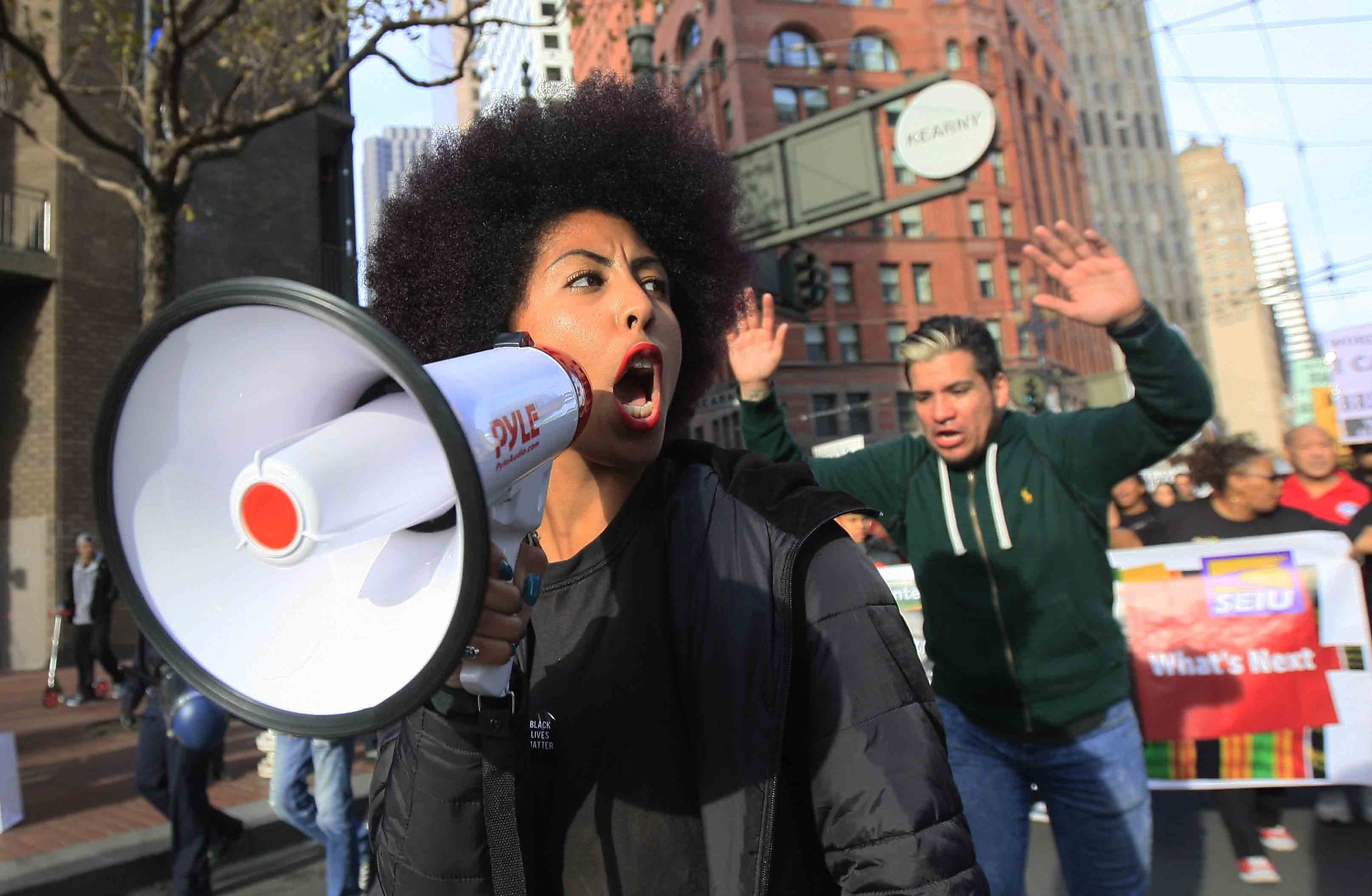In this striking daytime photo of a protest, a light-skinned African-American woman with a large, fluffy afro commands attention in the foreground. Dressed in all black and sporting red lipstick, she yells passionately into a white megaphone with red accents and a logo that reads P-Y-L-E, which she holds in her right hand, angled toward the bottom left of the image. Her head is turned to the right, her mouth wide open as she amplifies the protest's message. Behind her, a man in a green hoodie and blue jeans raises his hands in the air, perhaps echoing the "hands up, don't shoot" chant common in Black Lives Matter protests. He has black hair with a distinctive blonde streak. Marching alongside him and extending into the distance, a diverse crowd of African-American individuals and others hold a large banner, adorned with vibrant African cloth patterns in orange, green, and black designs, displaying the phrase "What's Next?" The protest unfolds on a cloudy day in a downtown cityscape, with tall buildings and distant onlookers on the sidewalk, all contributing to the powerful atmosphere of the demonstration.